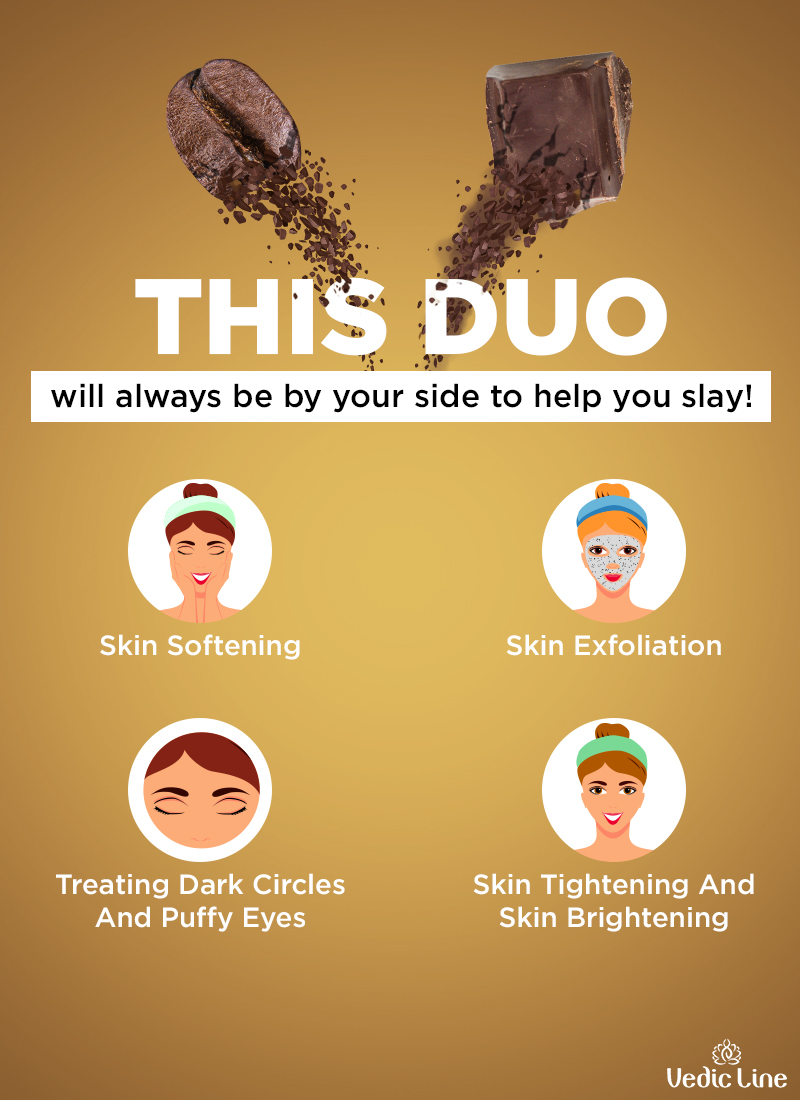**Discover the Perfect Duo for Radiant Skin**

This vibrant digital advertisement features a golden-yellow background that subtly fades to a darker shade at the top and bottom corners, creating a warm and inviting atmosphere. At the top left of the ad, an image of a coffee bean being crushed suggests vigor and freshness. Mirroring this on the right, a piece of chocolate being crushed evokes indulgence and luxury.

In bold, large, white capital letters, the headline powerfully states: "THIS DUO WILL ALWAYS BE BY YOUR SIDE TO HELP YOU SLAY." Beneath this promise, the narrative continues in smaller black font, further emphasizing the product's commitment to skincare excellence.

Four animated white circles arranged in two rows below the text highlight different skincare activities performed by women. From left to right, the circles depict:
1. Skin softening
2. Skin exfoliation
3. Treating dark circles and puffy eyes
4. Skin tightening and brightening

A logo and the words "Vedic Line" are strategically placed at the bottom right corner, reinforcing the brand identity and inviting viewers to embrace their path to flawless skin.